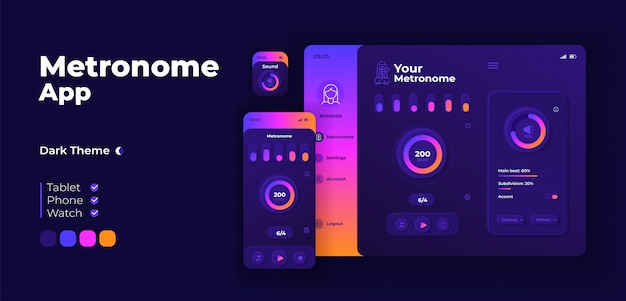The advertisement features a Metronome app displayed against a very dark, midnight blue background. Bold white text at the top left reads "Metronome App," followed by smaller white text that says "Dark Theme" accompanied by a crescent moon icon. Beneath, a bulleted list with purple and white checkboxes states the app's compatibility with tablet, phone, and watch. The advertisement showcases the app's dark-themed user interface with a central dial to adjust metronome speed and additional dials for timing settings. The mockups on the right illustrate the app on a watch, phone, and tablet, all adhering to the color palette shown in four rounded squares to the bottom left—dark violet, blue, pink, and yellow. Gradient navigational bars transition from goldish-yellow to pink to blue, complementing the dark violet backgrounds and uniformly colored elements across all device screens.